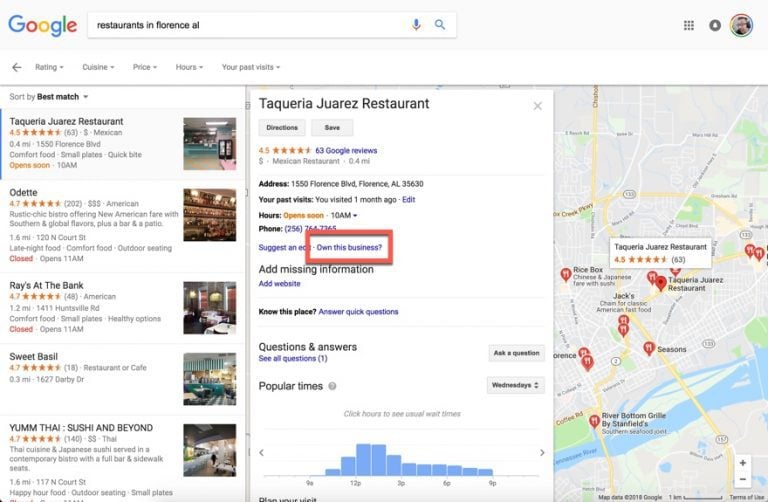Screenshot of a computer search results page on Google displaying restaurants in Florence, Alabama, sorted by best match. The top of the screen features the search query "restaurants in Florence, Alabama," along with a microphone icon for voice input and a magnifying glass for search. The page highlights five restaurants, all rated five stars. 

The first restaurant on the list is "Tequila." The details for "Tequila" are broad, covering various types of cuisine, including Mexican, Thai, sushi, and beyond. A map with pins indicates the locations of these restaurants. Specific information for "Tequila" includes its address, past visits, operating hours, phone number, and an option to add missing information. Additionally, it shows popular times to visit and a prompt in a red rectangle box with "Own this business?" followed by a question mark. The restaurant has garnered 63 Google five-star reviews. There is also a Q&A section for customer inquiries.

This detailed breakdown provides an in-depth look at the search results, highlighting the comprehensive information available for each listed restaurant.